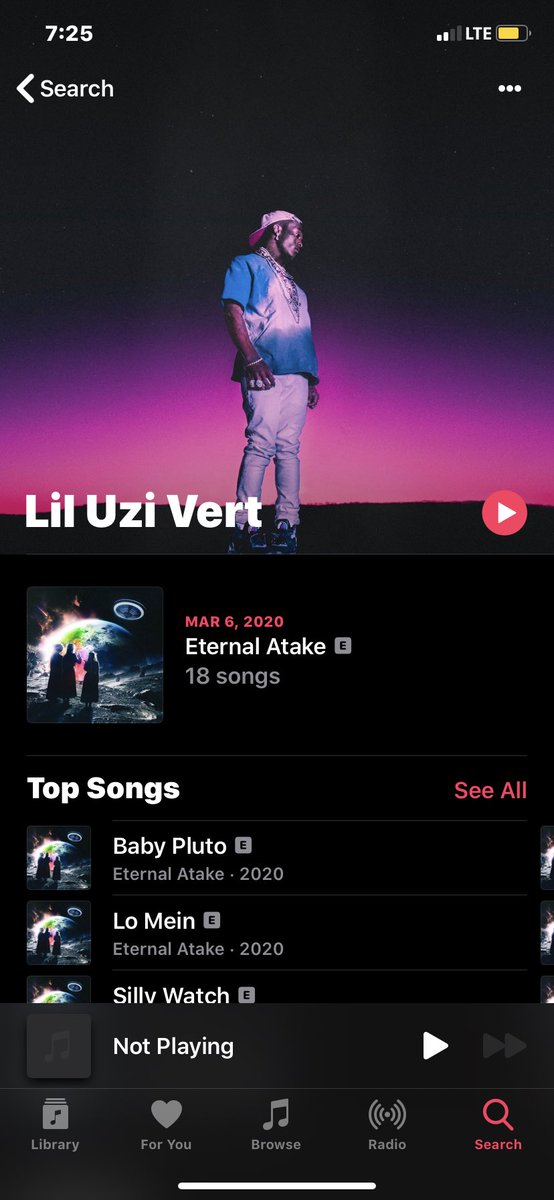In the 'Websites' category, this descriptive caption features a snapshot of a smartphone screen captured at 7:25, though it does not indicate AM or PM. The phone is connected to LTE, and the battery level is about 75% full. At the top of the screen, there is a search bar with a back arrow and three vertical dots adjacent to it. 

The background transitions from a dark hue at the top, gradually lightening from black to purple, then pink, and finally to a pale pink at the bottom. 

In the center of the screen stands an African American male with a baseball cap worn backward. He is dressed in a blue shirt paired with blue jeans. The screen prominently displays the name "Lil Uzi Vert" alongside a play button. Beneath this, it shows the release information: "March 6, 2020, Eternal Atake, 18 songs."

The visual element includes an image of people standing on Earth and gazing out at other planets from a spaceship vantage point. 

Below this image, the top songs listed are "Baby Pluto," "Lomane," and "Silly Watch," followed by the text "Not Playing." 

At the bottom of the screen, there is a navigation bar with the options: "Library," "For You," "Browse," and "Search."